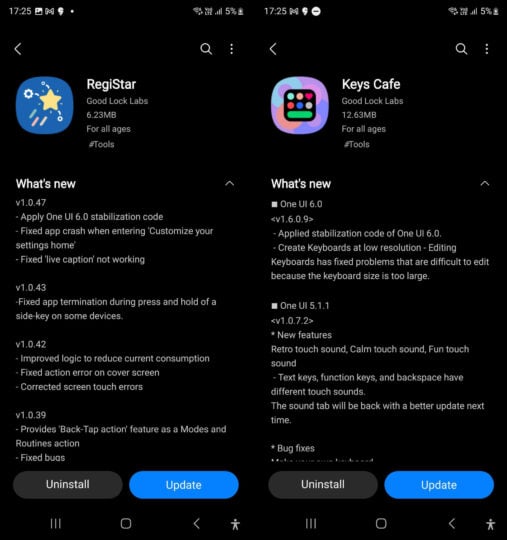This image features two side-by-side screenshots of app store pages showcasing recent software updates for two different apps. The background of both screenshots is black, with white text providing clear contrast and readability. 

On the left, we have a page for the app "Registar," developed by GoodLuckLabs. The app’s icon is a square with rounded edges, featuring a blue background and a prominent star. At the top, bold white text reads "What's New?" followed by a list of updates and version changes. One of the noted updates is for version 1.6.0, which includes "Stabilization Code." Towards the bottom of this page, there are two buttons: a gray "Uninstall" button and a blue "Update" button.

On the right, there is a similar setup for the app "Keys Café." The icon for Keys Café is visually distinct with a variety of colored squares, circles, and hearts. Like the Registar page, this screenshot also begins with the bold heading "What's New?" detailing the latest updates in the app’s software versions. Mirroring the left-hand screenshot, the bottom of this page also features a gray "Uninstall" button and a blue "Update" button.